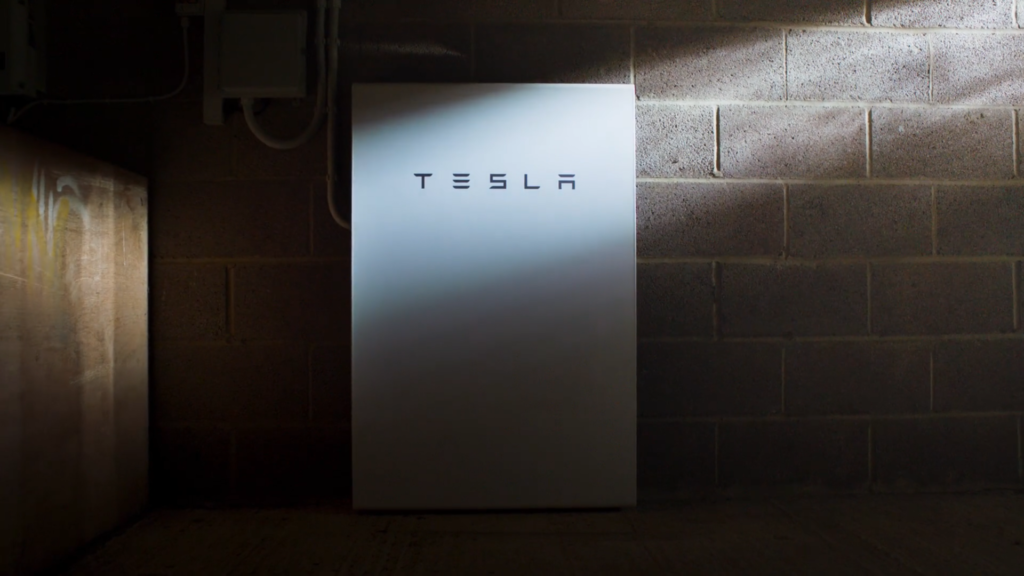A dimly lit image reveals a brownish-red brick wall with light subtly peeking through, illuminating the scene. Centered prominently is a white rectangle featuring the iconic Tesla logo, with "TESLA" written in silver-gray capital letters. Notably, the "E" lacks its vertical bar connecting the three horizontal lines, and the "A" appears slightly disjointed, characteristic of Tesla's unique typography. To the left of the logo, a closed brown door is visible, its surface marked with white spots, scratches, and signs of damage, adding a rugged contrast to the sleek, modern emblem at the center.